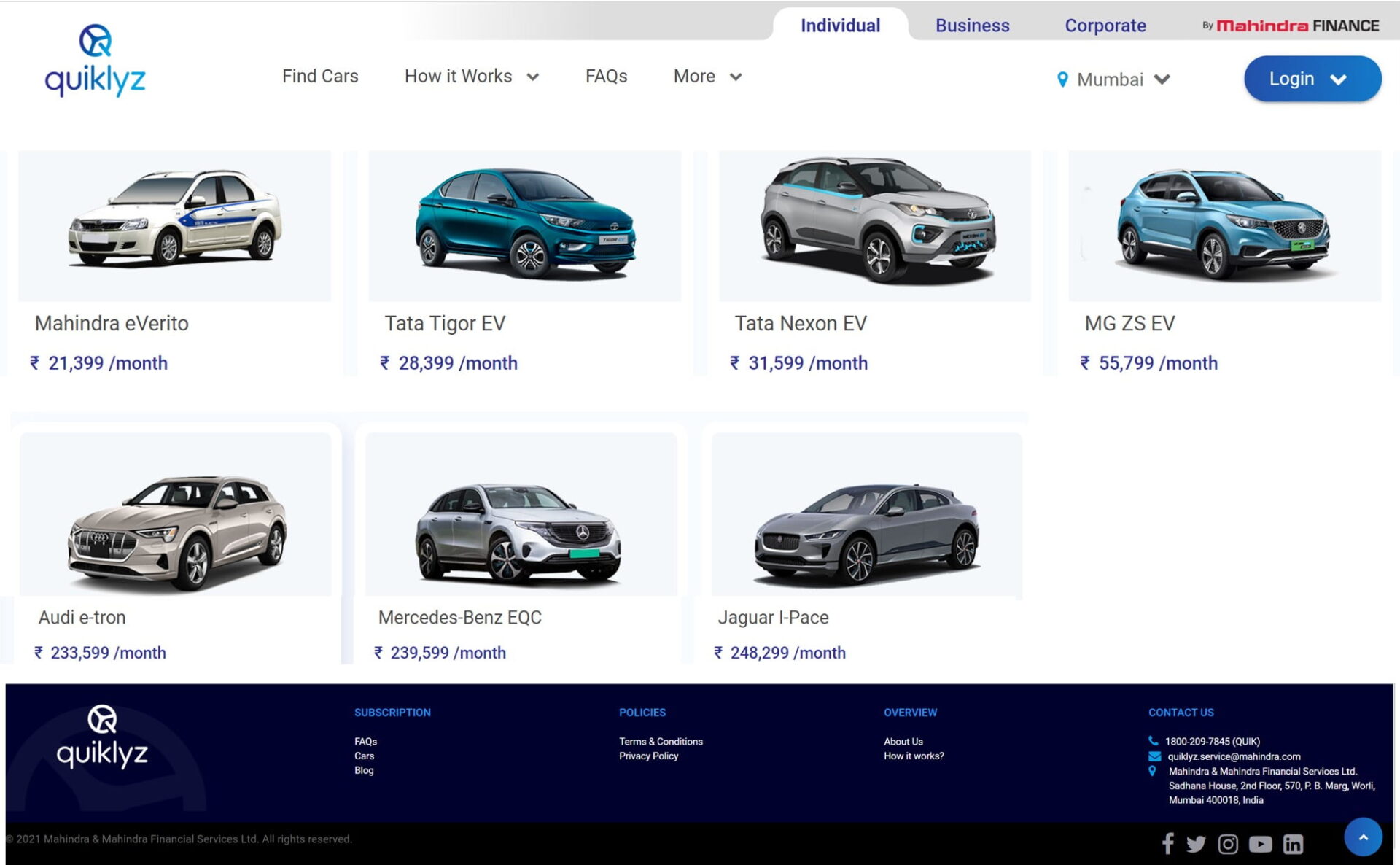This is a screenshot of a computer screen displaying a car sales website called "Quicklyz," identifiable by its two-tone blue logo featuring a steering wheel symbol. The website appears to cater to various customer types, offering options for individual, business, and corporate buyers. The main section of the screenshot showcases an array of seven cars, organized in a grid with four cars in the top row and three in the bottom row.

In the upper left, the Quicklyz logo is prominent, followed by the main content area where users can choose between different types of buyers. The selected option seems to be "Individual."

Detailing each car, starting from the left:
1. A white Mahindra e-Verito with a blue stripe down the side, priced at $21,399 per month.
2. A bright teal blue Tata Tigor EV, priced at $28,399 per month.

The displayed cars include their names and monthly prices, providing a clear and concise view for potential buyers browsing the website.